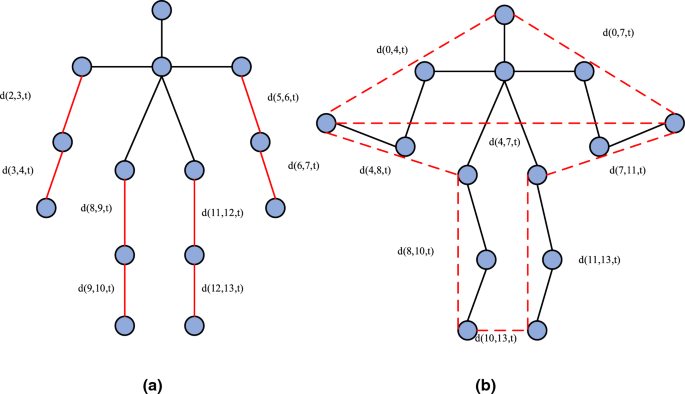The image consists of two separate charts labeled (A) and (B). Both charts resemble flowcharts, featuring blue circles interconnected by thin black lines. In Chart A, a single blue circle at the top splits into three more blue circles, which branch out further, each labeled with combinations like D, 3, 4, T, D, 11, and 12. Chart B mirrors Chart A in structure but includes a red perforated line outlining and pointing upwards, suggesting boundaries or movement constraints. Both charts are devoid of any titles or explanations, hinting at their use in something like CGI modeling, where one chart depicts the basic structure and the other outlines the possible extents of movement.